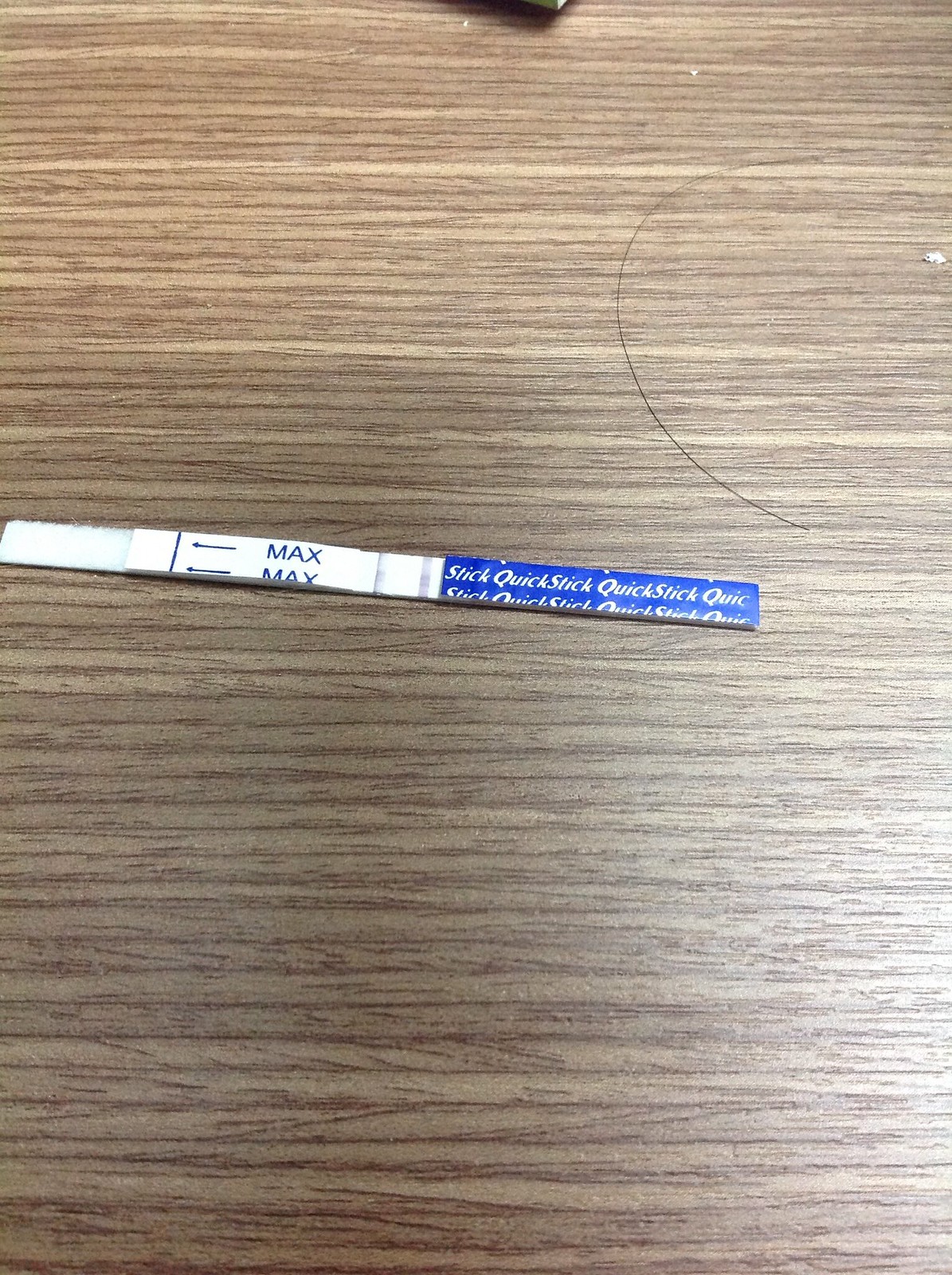The image showcases a QuickStick drug test laying on a grayish wooden table. The test strip is positioned predominantly on the left-hand side of the image, with the portion designed to be dipped into a urine sample extending to the edge of the frame. The drug test strip is composed of three distinct sections: the first is a large, cotton-like area that comes into direct contact with the urine sample; adjacent to this is a paper segment featuring a black line accompanied by two arrows pointing towards it, and the word "MAX" printed twice in capital letters, one above the other. The final section to the right of this consists of a blue background adorned with the white text "QUICKSTICK." Above the QuickStick test on the wooden table, there is a small hair follicle alongside what looks like dandruff or dust particles.